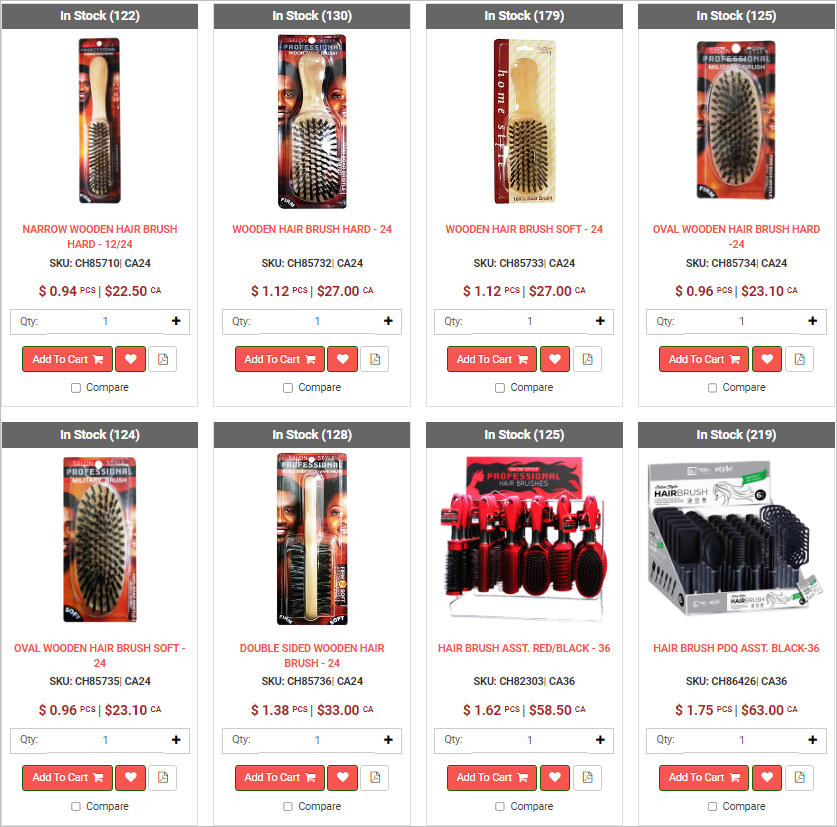This screenshot depicts a product page from a website featuring two rows of hairbrushes, each row containing four items, totaling eight products. The majority of the hairbrushes are wooden with large black bristles. Each brush is presented in a vertically oriented rectangle that includes detailed information such as the product name, SKU, and price, with prices ranging from $0.94 to $63.00. Additionally, there are controls for selecting quantity, adding to cart, favoriting, comparing products, and an unidentified button that resembles a piece of paper with a folded corner.

The top row showcases a variety of wooden hairbrushes: from a thin and thick brush on the left to a smaller and oval-shaped brush on the far right. The bottom row continues with diverse styles, including a long oval brush on the far left, a dual-sided brush next to it, and two plastic brush sets in red and gray. The latter also appears to include a professional kit and a cardboard box filled with additional hairbrushes and display products on the bottom right. Several product labels feature smiling faces of a black man and woman, enhancing the visual appeal. Each item listing also displays the stock quantity available from the retailer.